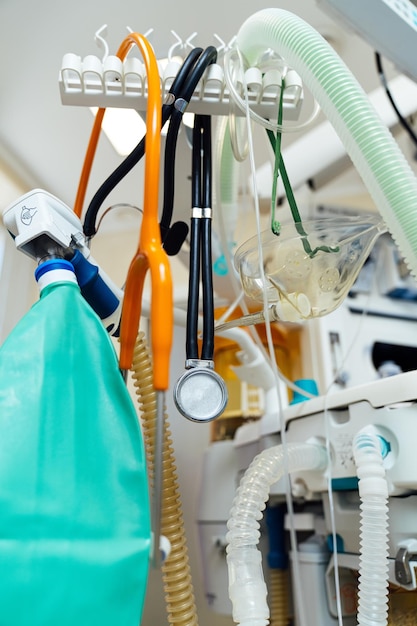This close-up image presents a detailed array of medical tools and equipment commonly found in a doctor's office or operating room. Central to the composition is a white rack, from which numerous tubes and instruments are suspended, including an oxygen face mask attached to one of the tubes. Prominently visible on the left side is a turquoise, inflatable bag with a nozzle, likely used in ventilation. Next to it, an orange stethoscope and a black stethoscope are neatly hanging, showcasing the variety in color and texture among the instruments. The right side features several clear and light green transparent tubes, attached to a machine that remains partially out of view. The background is purposefully kept empty, directing all attention to the medical equipment displayed.